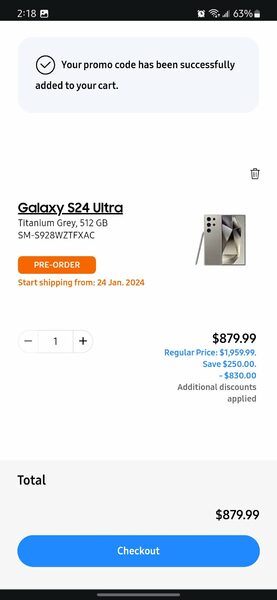Screenshot of a mobile shopping app displaying the purchase details for a Galaxy S24 Ultra phone in Titanium Gray. The screen highlights a significant discount; the original price of $1,959.00 has been reduced to $879.99, thanks to a $250 discount and an additional $830.00 off. At the bottom of the screen, there is a prominent orange "Pre-Order" button, encouraging users to secure their purchase ahead of time. Below this button is a blue "Checkout" button, ready for the user to finalize the transaction for this high-end device.